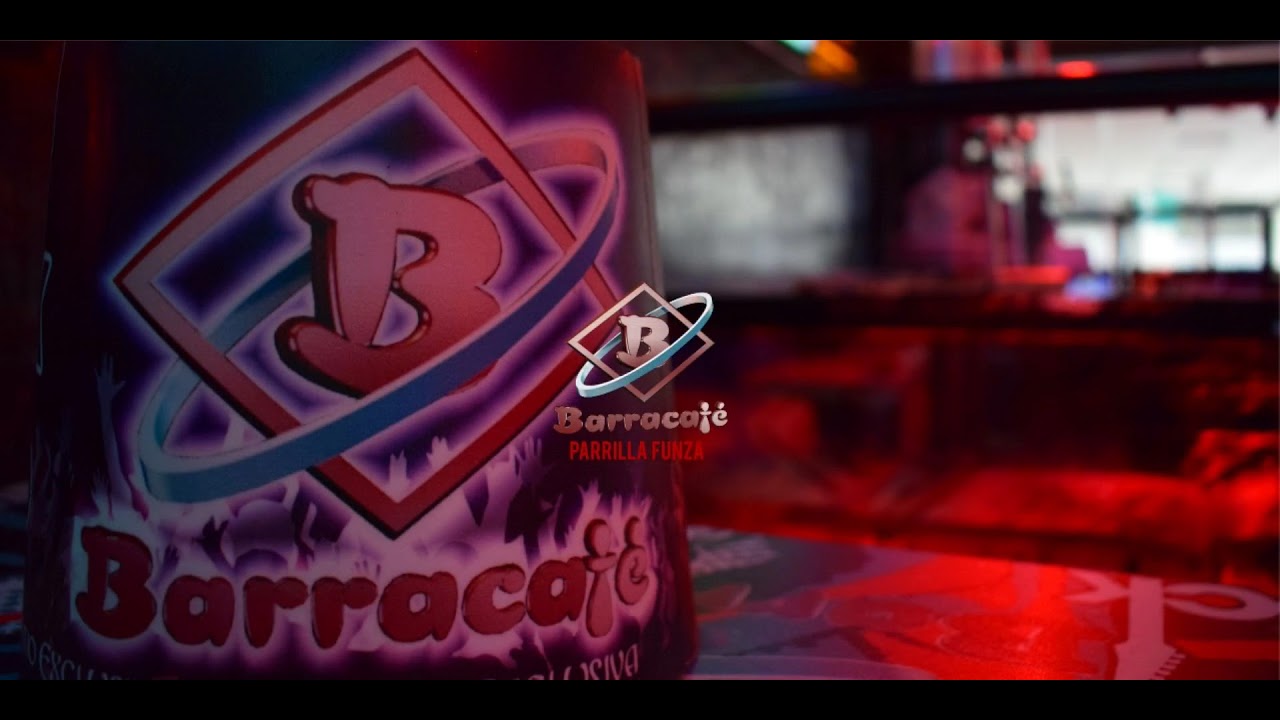The image appears to be a publicity photograph for a venue, presumably a restaurant, bar, or club, characterized by its dim and reddish lighting. Dominating the left side is a close-up of a branded object featuring a white capital 'B' inside a white square tilted at an angle and surrounded by a blue ring. Below the logo are the words "Barra Cafe" and "PARRILLA FUNZA" in red capital letters. The same logo and text are superimposed prominently at the center of the image, which has an overall blurred background that likely represents the interior of the venue, with hints of tables, chairs, and possibly a person. The object with the logo includes a colorful print comprised of reds, blues, whites, and purples, adding visual interest.